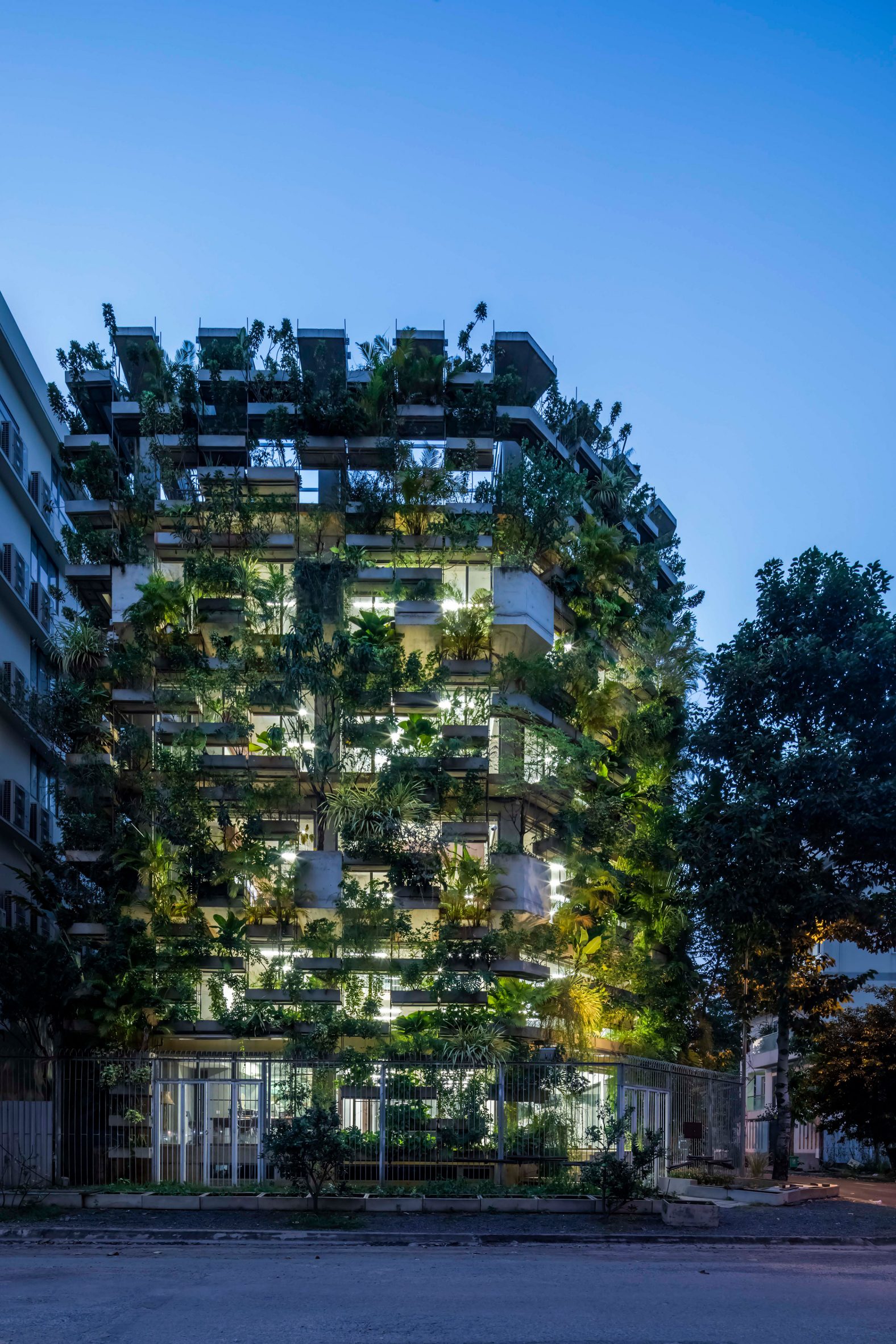This photograph captures a strikingly unique, multi-story modern building almost entirely covered in lush, thriving plants. The structure, which stands about six levels tall including the rooftop, features an abundance of greenery spilling over from its numerous terraces and balconies, giving it the appearance of being enveloped by nature. Each floor showcases diverse plant life, creating a vertical garden that contrasts beautifully with the building’s sleek design.

On the ground level, a thin silver fence or possibly a white one runs along the sidewalk, adding to the urban setting while preventing trespassing. To the right of the building stands a dark, tall tree, and in the background to the right, a smaller white building is visible along with additional trees. The left side of the photo reveals a glimpse of an adjacent building that resembles the main structure in color.

The street in front of the building appears empty and ready for traffic. The time seems to be around dusk, with a clear blue sky overhead, suggesting either sunset or nightfall. Some artificial lights are on inside the building, adding a warm glow to the scene. The combination of urban architecture and flourishing plant life creates a captivating, almost surreal visual that hints at an artistic or environmentally-conscious design.